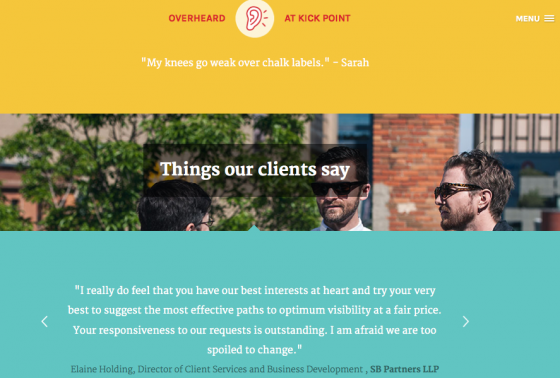The website features a structured layout divided into three distinct horizontal sections. At the top, a gold banner prominently displays the heading "Overheard at Kick Point," accompanied by an icon of a circle with an ear and radiating lines, symbolizing the act of overhearing. To the right of this banner, a navigation menu and a hamburger icon provide easy access to different parts of the website.

Beneath the gold banner, another section features the quote: "My knees go weak over chalk labels. - Sarah." Below this, in the middle section, there's an image of three men engaged in conversation outdoors, possibly between buildings with a tree in the background. This image is overlaid with the caption "Things our clients say," suggesting that the men are listening and possibly sharing their experiences.

The bottom third of the website is in a light teal color and contains a paragraph of text, center-justified, praising the company's services. The testimonial reads: "I really do feel that you have our best interests at heart and try your very best to suggest the most effective paths to optimum visibility at a fair price. Your responsiveness to our requests is outstanding. I'm afraid we are too spoiled to change." This section also features navigation arrows allowing users to browse through various client testimonials.